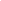Detailed caption:

The image depicts a sophisticated real estate search tool interface, prominently featuring a comprehensive map and a detailed list of property listings. At the top of the interface, there is a search bar labeled "Name This Search" that also provides suggestions such as Newport Beach, condominium, and closed properties. Each property listing is displayed in detailed cards that feature essential information including the address, city, price, status (e.g., closed), number of bedrooms and bathrooms, square footage, and days on market (DOM). 

Embedded within the cards are thumbnail images of the respective properties, providing a visual preview. The map also showcases the property locations marked with price tags for quick reference. Highlighted properties include:
- 2402 Santa Ana Avenue #8, Newport Beach, CA, priced at $630,000 and marked as closed, featuring 2 bedrooms and 4 bathrooms.
- 210 Orange Street, Newport Beach, CA, priced at $1,412,500 with 2 bathrooms and 1,390 square feet of living space, noted as an impressive listing.
- 7 Bartholomew Court #19, Newport Beach, CA, listed at $840,000, with details unspecified.
- 79 Corsic Drive, a unique listing priced at $30,450 and marked as closed, with unclear additional details, possibly the reason for the screenshot being taken.

Overall, the image provides a clear and structured overview of available and recently closed real estate properties, intended to assist users in their property search.